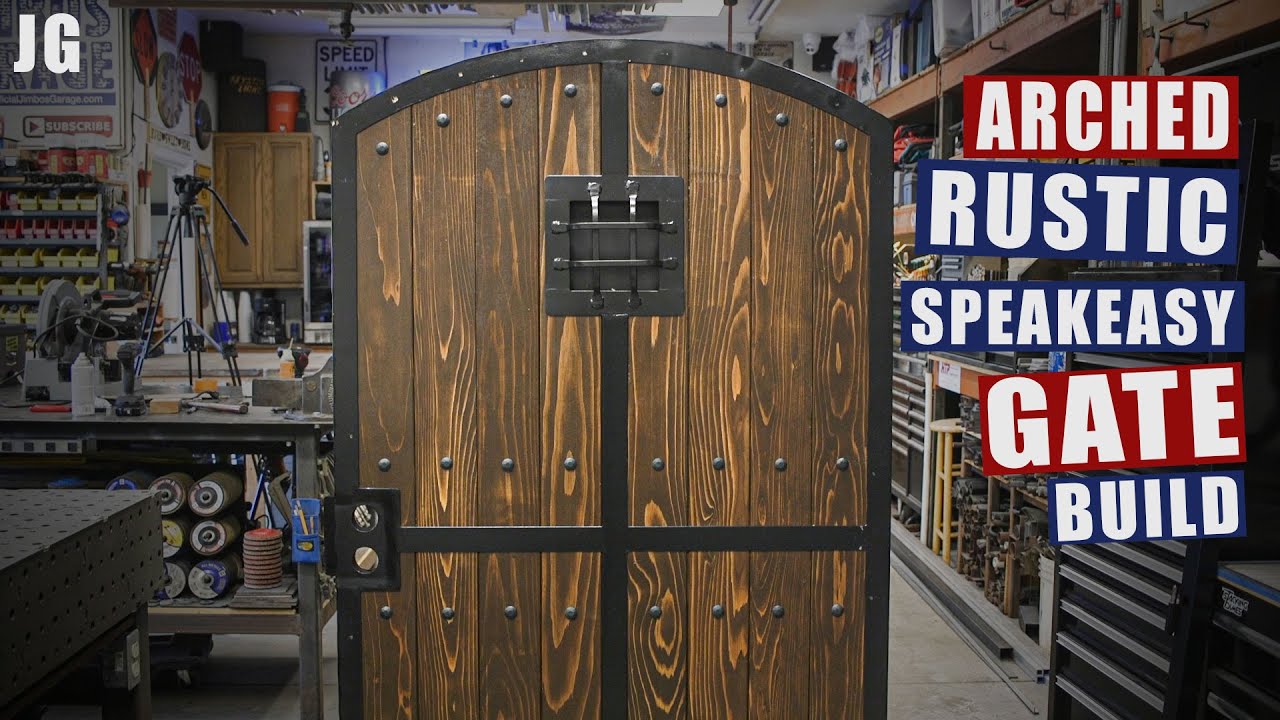In the foreground of the image, a robust, studded, dark wooden door dominates the scene, framed by black borders and reinforced by silver metal studs meticulously arranged along the top, middle, and bottom sections. The door is sectioned by black metal brackets intersecting horizontally and vertically, overlapping and adorned with studs both above and below these brackets. Slightly above the middle of this formidable door is a small barred window designed to slide open from the inside, conveying a sense of both utility and strength. 

In the background, the scene transitions to a busy wood workshop or construction studio, filled with an array of woodworking tools, saws, paints, counter space, drawers, electronics, stools, and various other equipment. The backdrop features white walls, floor-to-ceiling shelves packed with a variety of items, a speed limit sign, and light brown wooden door shelves. A silver island table with a black tripod on it, as well as several round canisters underneath, further clutter the environment. 

The right side of the image is marked with segmented bars of white text on red and blue backgrounds, sequentially reading "Arched," "Rustic," "Speakeasy," "Gate," "Build." Additionally, the upper left corner prominently displays the initials "JG" in white capital letters, adding a final touch of detail to the intricate setting.